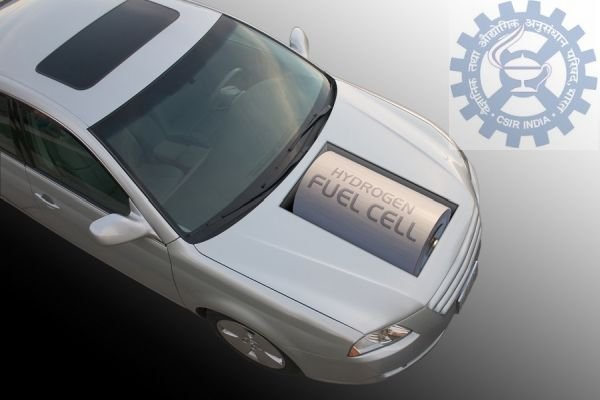This image features a highly detailed, computer-generated model of a silver, four-door sedan, viewed from a top-down angle. The car boasts a visible sunroof and prominent front windshield through which the interior, including the seats, can be seen. The most striking feature of the car is the large, gray hydrogen fuel cell prominently displayed in a cutout area on the hood, indicating its eco-friendly technology. The background of the image transitions from light gray in the upper right corner to dark gray, almost black, in the bottom left, creating a dramatic contrast. In the upper right corner, there's a logo featuring a circular gear with spokes, surrounding an old-style lamp, accompanied by the text "CSIR" and "India" in white. The emblem is rendered in light blue and white, with additional text in a foreign script around its border, enhancing the sophisticated and promotional nature of the piece.